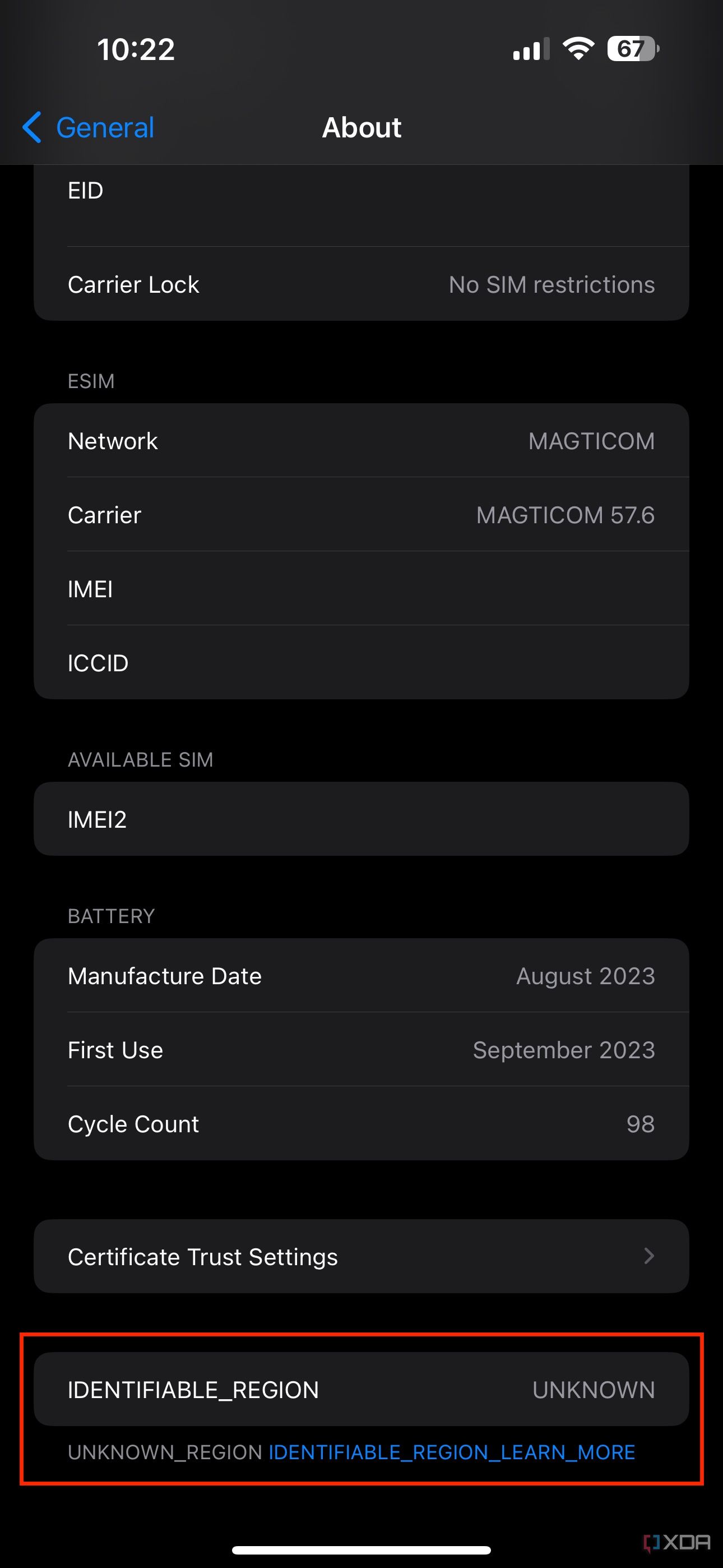Here’s a detailed and cleaned-up version of the descriptive caption:

---

This image is a screenshot of the "General" section of a smartphone, either an iPhone or Android device. The background is black, and the word "General" appears prominently in blue at the top, next to an arrow indicating a back button. The phone's status bar shows it is 10:22 AM, and the battery is at 67%.

Below the "General" heading, the first item listed is "About," written in white text. Under this, there is a section labeled "EID," followed by "Carrier Lock," showing "No SIM restrictions." The details pertaining to network information are "eSIM Network - Mag-to-Com" with "Carrier - Mag-to-Com 57.6."

Further down, there are technical identifiers: "IMEI" followed by "ICCID," and the section titled "Available SIM" lists "IMSI." The next entry is "Battery," which provides manufacture and usage details: "Manufacture Date - August 2023," "First Use - September 2023," and "Cycle Count - 98."

At the bottom, you see "Certificate Trust Settings" with an arrow indicating further options. Just above the bottom, there is a distinctive red rectangular box with "Identifiable Region" written in white text, showing "Unknown" for both region and identifiable area. Lastly, there is text stating "Identifiable Region - Learn More."

---

This detailed caption provides a comprehensive description of every visible element on the screen.